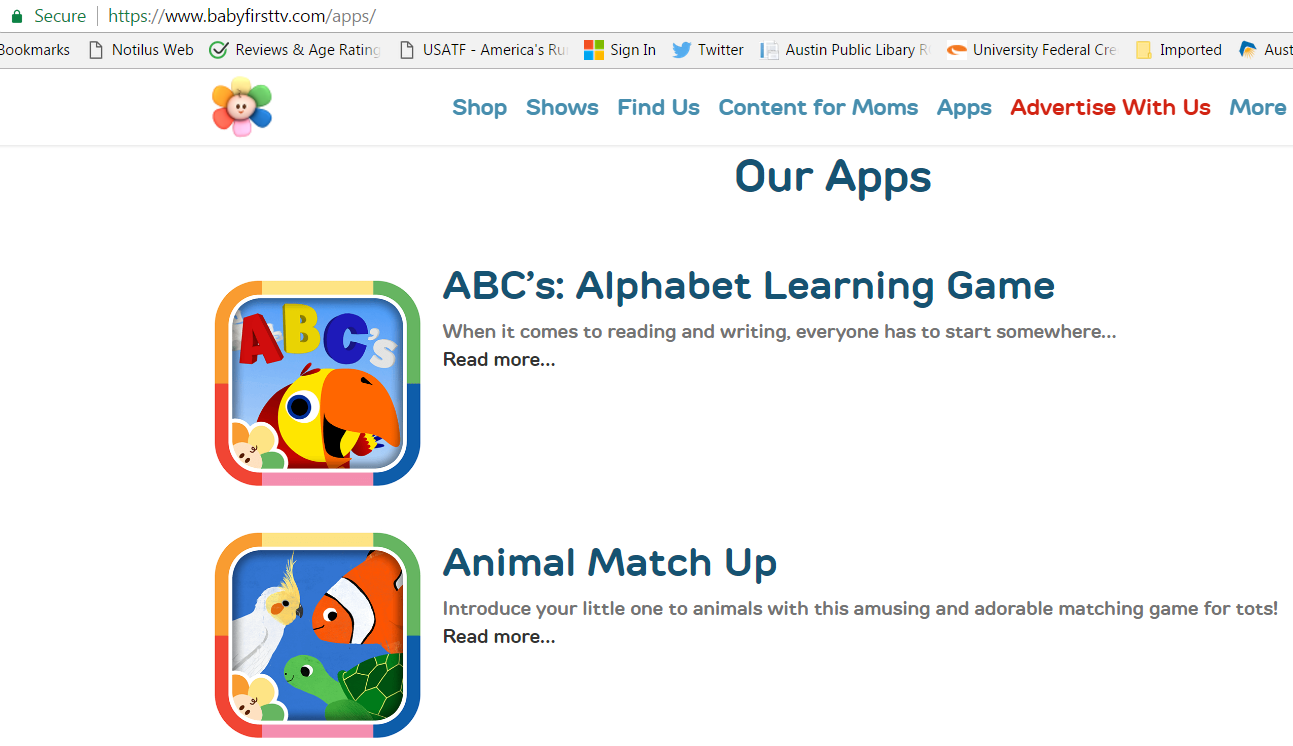This screenshot captures a desktop view of the BabyFirstTV website at https://www.babyfirsttv.com/apps/. The specific browser used is not identifiable. Along the top of the browser, multiple bookmarks are visible including links to: Nautilus Web Reviews and Age Ratings, USATF America's [subject unspecified], Signing into Microsoft, Twitter, Austin Public Library, University Federal Credit Union (likely imported), and another Austin-related bookmark.

The main content of the webpage is centered around a cheerful flower with a smiling face and rainbow-colored petals. The navigation menu showcasing options reads from left to right in segments of blue and red: "Shop," "Shows," "Find Us," "Content for Moms," "Apps," "Advertise with Us," and "More."

Prominently featured on the page are two app promotions, each highlighted in vibrant frames gradating from yellow to green, blue, pink, red, and orange. The first app, named "ABCs Alphabet Learning Game," features an image of a multicolored parrot, with the text detailing the app's focus on beginner reading and writing. The description encourages further exploration with a "Read more..." prompt.

The second app, titled "Animal Matchup," is adorned with illustrations of an orange clownfish, a green turtle, and a lutino cockatiel. This game aims to introduce young children to various animals through a delightful matching experience. Similarly, it invites interested visitors to "Read more..."

Both apps are designed for babies and young children, emphasizing educational fun suitable for early learning stages.